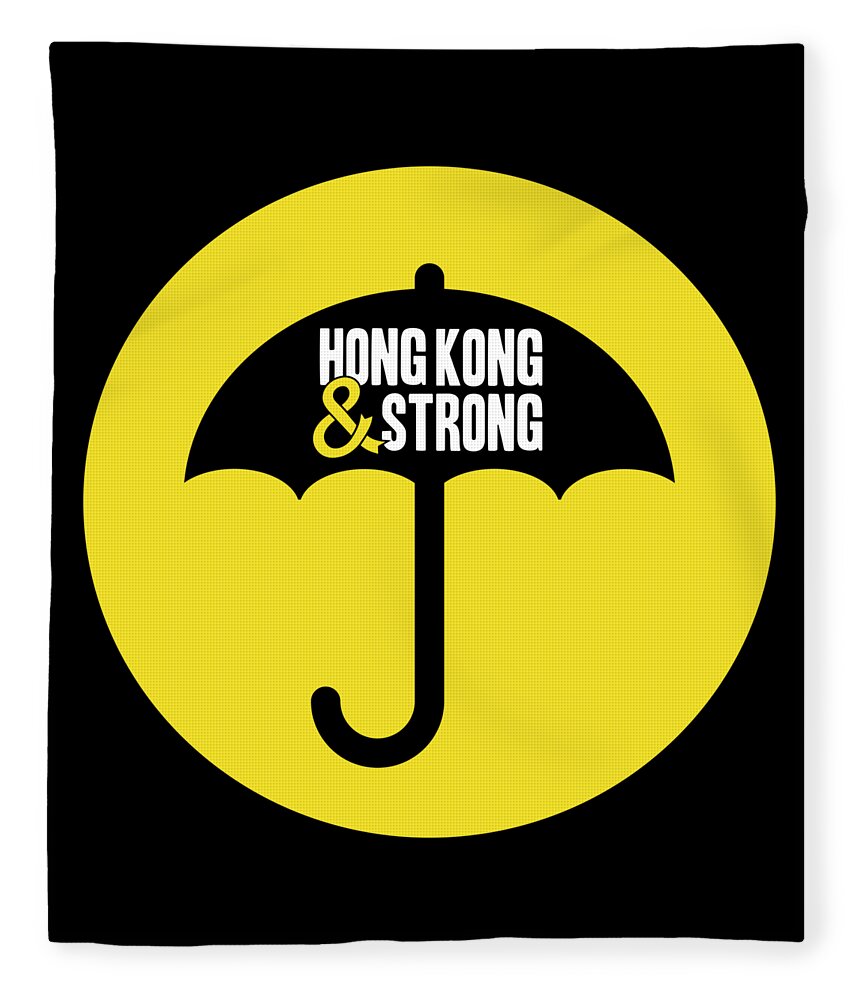This image features a logo set against a dark black background with slightly rounded corners, giving it an irregular, possibly blanket or banner-like border. Central to the design is a vibrant yellow circle, composed of slightly darker yellow pixel-like dots. Prominently displayed within this circle is the silhouette of an open black umbrella, characterized by its four-pointed bottom edge, a small rounded tip above, and a distinctive J-shaped handle. Overlaid on the sloped part of the umbrella are the bold white capitalized words "Hong Kong" and "Strong." These two words are separated by an ampersand symbol, uniquely fashioned to resemble a yellow ribbon. The strong contrast between the black and yellow elements enhances the visibility and impact of the central motif, suggesting a logo likely associated with a charitable cause or a significant movement.